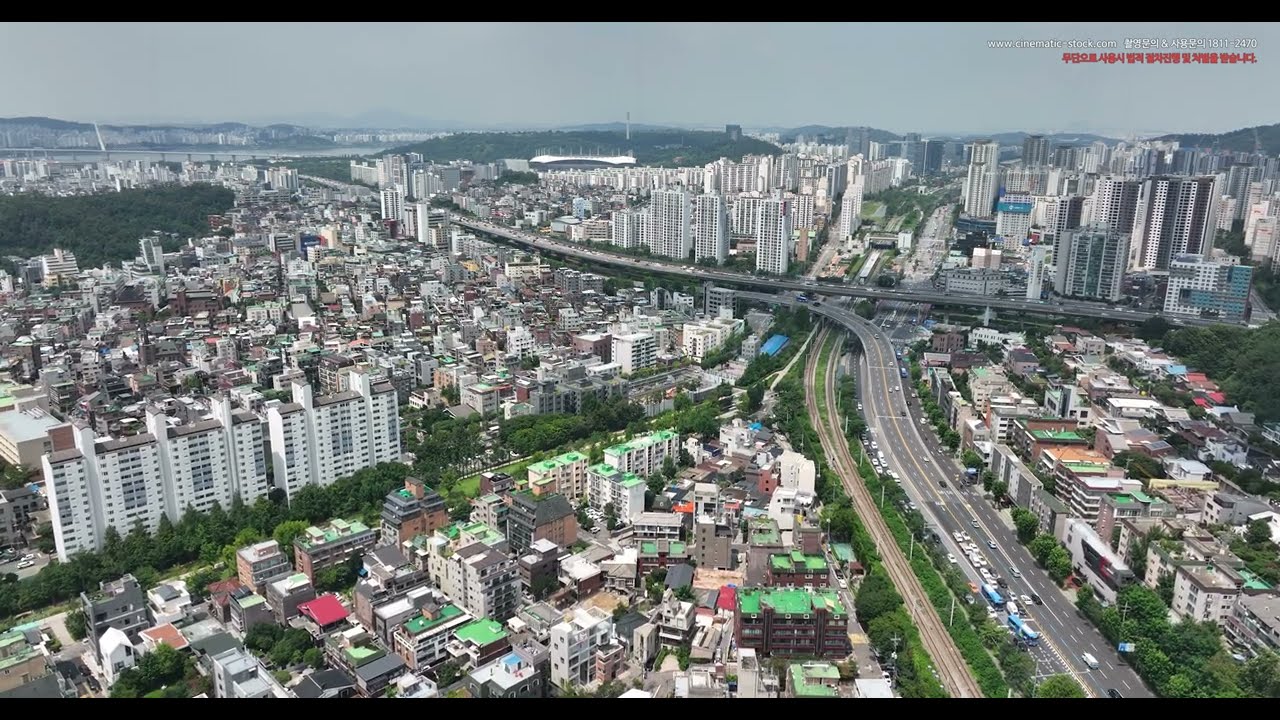The aerial photograph captures a sprawling metropolitan cityscape, characterized by densely packed high-rises and skyscrapers, with a large freeway slicing through the urban expanse. The freeway, a double-lane highway, runs from the bottom right of the image, curves toward the left, and continues to the upper left, illustrating the heavy traffic typical of a bustling metropolis. Near the center of the image, there is a prominent bridge structure, adding to the complexity of the transport network which also includes parallel train tracks suggesting efficient connectivity within the city.

On the right side, clusters of taller buildings with dotted windows dominate the skyline, some featuring distinctive green roofs, which appear unusual amidst the urban density. The left side contains slightly shorter buildings and a unique area of greenery, possibly a park, which stands out in an oval shape among the sea of concrete.

The photograph also captures the natural elements of the city backdrop with a mountainous skyline visible in the distance, giving context to the city’s geographical setting. The image has a watermark in Asian characters, likely indicating a Japanese or other East Asian city, with the website www.cinema-stock.com also visible, suggesting the source of the photograph. Despite the cloudy sky, natural sunlight enhances the detailed textures and elements of this highly populated and structured urban setting.